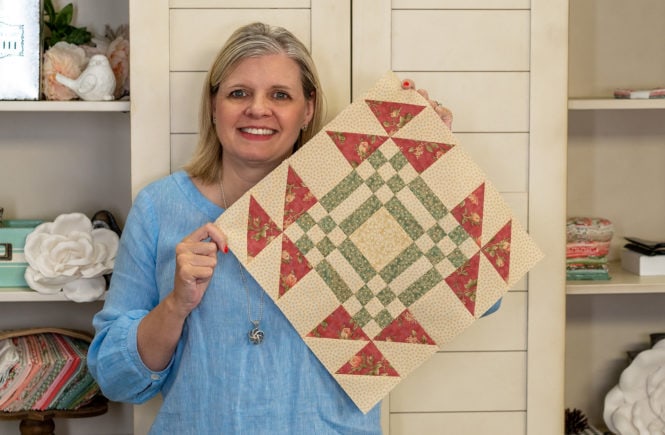In the image, a woman with blonde hair, parted on the side, is standing in front of an off-white cabinet with multiple shelves containing various folded items. She is wearing a blue, long-sleeved shirt and smiling as she holds up what appears to be a quilt square or a piece of material. The quilt square is approximately a foot across, featuring an intricate design. The border is adorned with orangish triangles, some decorated with floral patterns, and tan triangles. The inner section comprises a mix of green and white rectangular and square boxes forming a pattern, with a plain tan square featuring a few dots in the very center. Her right elbow is bent as she pinches the corner of the quilt square with her fingers, while her left hand holds the top corner. Behind her, the cabinet shelves house what seem to be linen supplies used for her quilting work.